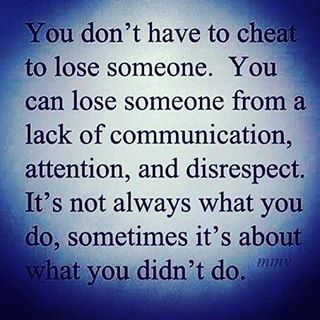The image is a poster with a blue gradient background that darkens towards the edges and lightens into a pale blue circle in the center. Across this circle, there is text in black font that reads: "You don't have to cheat to lose someone. You can lose someone from a lack of communication, attention, and disrespect. It's not always what you do. Sometimes it's about what you didn't do." The typography includes punctuation such as periods and commas, and there is a notable double space after the first sentence. In the lower right-hand corner, there are smaller italic blue letters spelling "MMY."